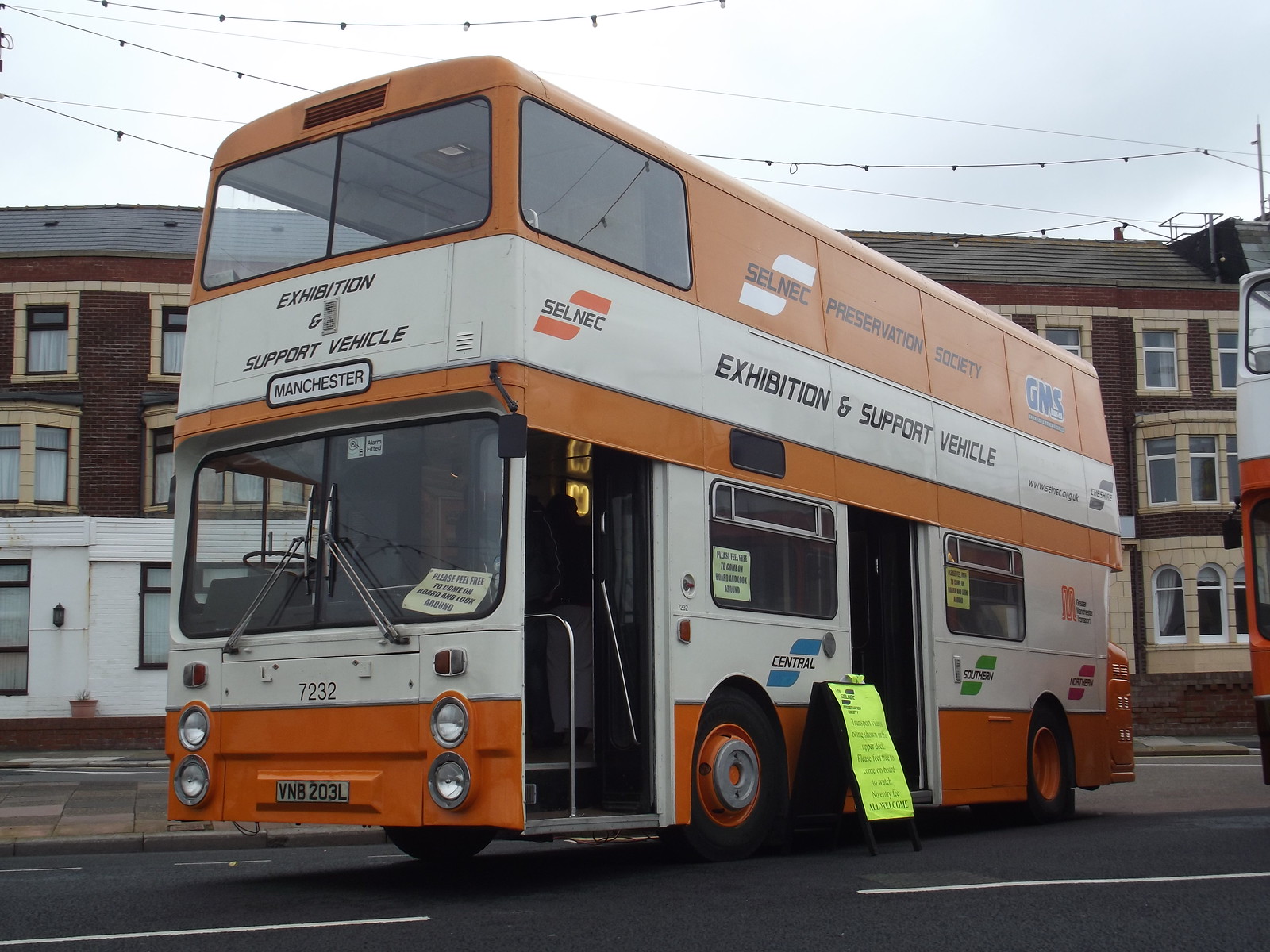This detailed photograph showcases an orange and white double-decker bus, prominently centered against a backdrop of multi-story brick row houses with white fronts and slanted roofs. The bus, viewed from its left side and slightly angled to the left, features an orange stripe at the bottom and another set around the top section. The area between these orange stripes is predominantly white. At the front, the bus displays "Exhibition and Support Vehicle Manchester" in bold black text. The windows include upper-level orange-bordered side windows, a front driver's window, and a lower section showing an entryway with a handrail. The bus carries the number 7232 and license plate V203 LB. Additional text on the side reads "Selnick Preservation Society Selnick Exhibition and Support Vehicle" with the website "www.selnick.org.uk" and locations "Cheshire, Central, Southern, Northern." Notably, a neon sign states, "Please feel free to come on board and look around," and another neon sign announces a transport video being shown on the upper deck. The bus resides on a gray road with white lines, under a gray cloudy sky outlined by power lines. In the background, amid the row houses, there’s a sliver of another double-decker bus, suggesting the setting is a bus exhibition. The photograph emphasizes the vibrant colors of orange, white, and additional highlights of black, neon yellow, brown, and gray, encapsulating a nostalgic, informative, and inviting atmosphere.